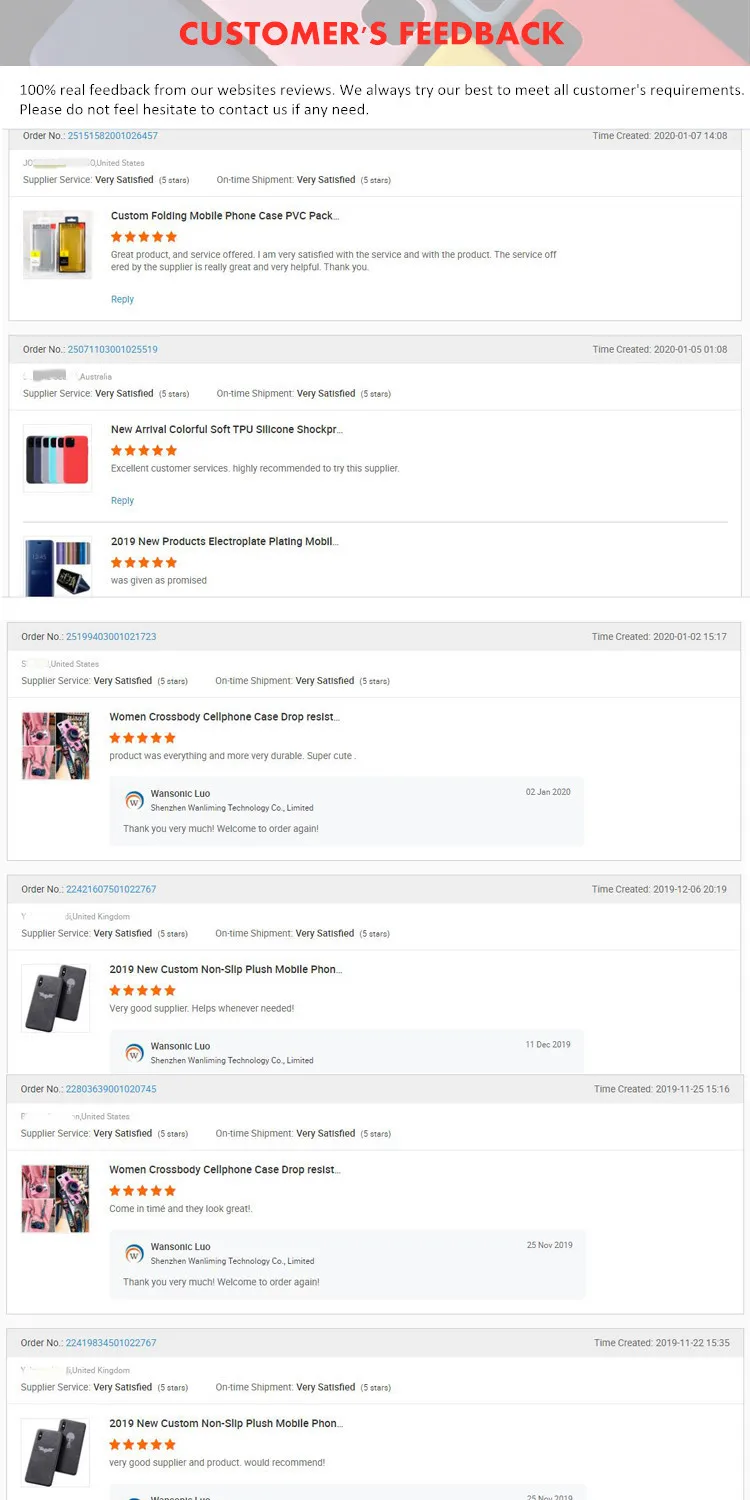**Detailed Caption:**

The screenshot depicts the backend interface of an e-commerce website, showcasing authentic customer feedback on various products. The heading clearly states "Customer's Feedback: 100% Real Feedback on Our Website's Reviews." It emphasizes the company's commitment to meeting all customer requirements and encourages customers to reach out if they have any needs.

1. **Custom Folding Mobile Phone Case, PCPVC Pack:**
   - **Rating:** ★★★★★
   - **Review:** "Great product and service offered. I'm very satisfied with the service and the product. The service offered by the supplier is really great and very helpful."

2. **New Arrival Colorful Soft TPU Silicone Shock (partial view):**
   - **Rating:** ★★★★★
   - **Review:** "Excellent customer services. I highly recommend trying this supplier."

3. **2019 New Products Electroplate Plating Mobile (ambiguity in product, possibly a phone stand):**
   - **Rating:** ★★★★★
   - **Review:** "Was given as promised."

4. **Women Cross-Body Cell Phone Case Drop Resist:**
   - **Rating:** ★★★★★
   - **Review:** "Product was everything and more. Very durable, super cute."
   - **Seller's Response:** "Thank you very much. Welcome to order again."

5. **2019 New Custom Non-Slip Plush Mobile Phone Case:**
   - **Rating:** ★★★★★
   - **Review:** "Very good supplier. Helps whenever needed."
   - **Seller's Response:** "Shenzhen Wen Lending Technology Company Limited" (Note: the response is partially cut off.)

6. **Women Cross-Body Cell Phone Case Drop Resist (another instance or repeated product):**
   - **Rating:** ★★★★★
   - **Review:** "Came in time and they look great."
   - **Seller's Response:** "Thank you very much. Welcome to order again."

7. **2019 New Custom Non-Slip Plush Mobile Phone Case (repetition):**
   - **Rating:** ★★★★★
   - **Review:** "Very good supplier and product. We recommend."
   - **Seller's Response:** (Partially cut off.)

Each review highlights a five-star rating, illustrating customer satisfaction with the products and the services provided by the supplier. The supplier's responses, although sometimes cut off, express gratitude and encourage future orders.